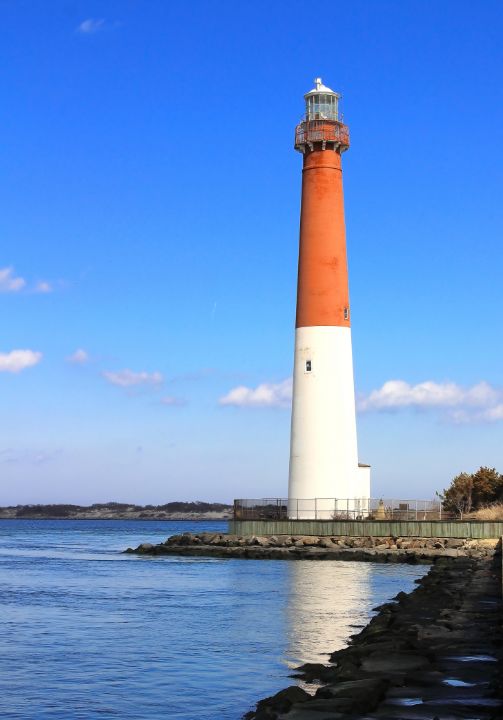The image is a color photograph taken during the day, showcasing an impressive lighthouse situated by the shore. The sky overhead is an expanse of vibrant blue, dotted with a few fluffy, white clouds that enhance the serene atmosphere. The lighthouse stands tall with its base painted a crisp white and the upper section a striking red. A white roof caps the top where the light is housed. Surrounding the base of the lighthouse is a sturdy fence, likely around 10-12 feet tall, designed to keep people out.

In front of the lighthouse, rocky shores meet the water, creating a rugged and picturesque coastline where waves crash energetically against the rocks. The water reflects the distinct colors of the lighthouse, adding to the scenic beauty of the image. Visible within the lighthouse structure are two small, square windows - one on the white lower section and the other on the red upper section.

To the right of the lighthouse, there are a few trees, adding a touch of greenery to the predominantly rocky landscape. Further in the background, rolling hills or small mountains rise up, enhancing the natural setting. The photograph captures both the majesty of the lighthouse and the tranquil yet dynamic interaction between the land and sea.